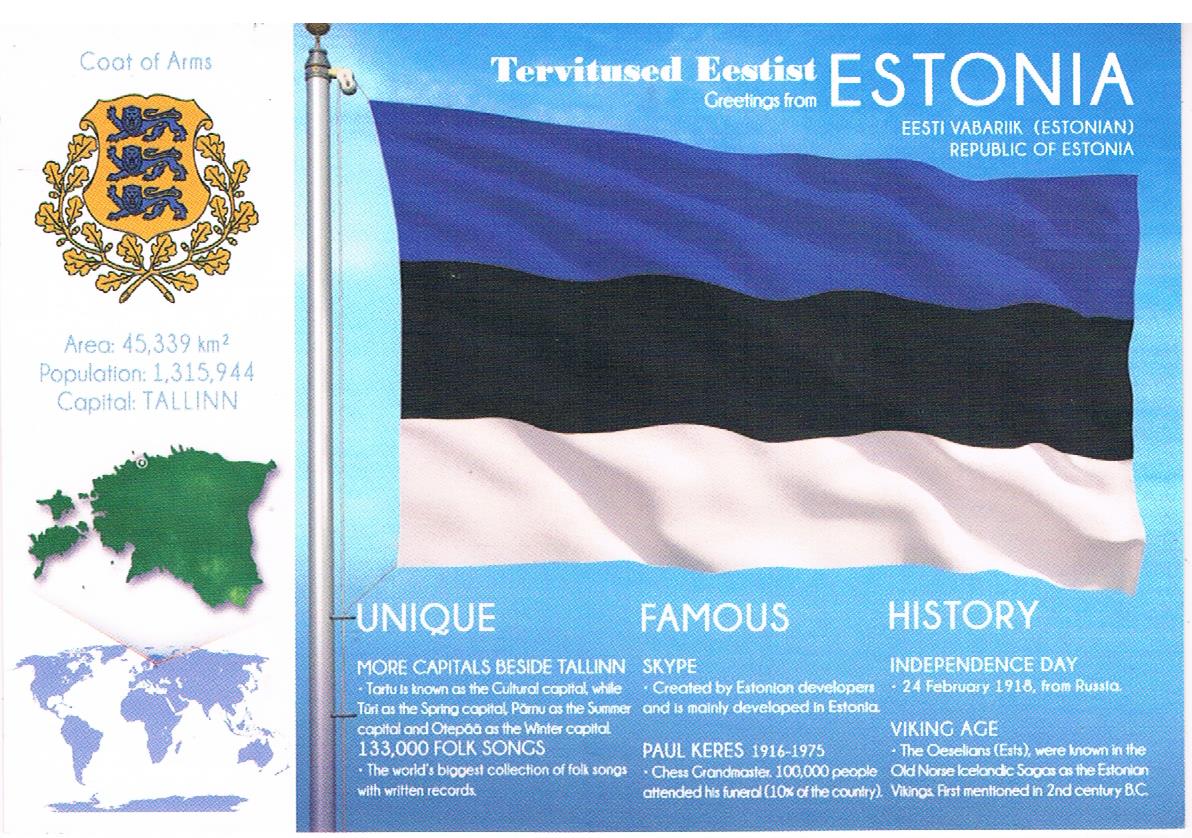The digitally generated rectangular image showcases an informative ad about Estonia against a striking light blue background. Dominating the center is the flag of Estonia, fluttering from a silver pole. The flag features three horizontal stripes: dark blue at the top, black in the middle, and white at the bottom. Above the flag, the text reads "Tervitus Estis," alongside "Greetings from Estonia" and "Republic of Estonia." Below the flag, three subheadings—Unique, Famous, and History—provide detailed facts about the country. 

The left side of the image features a vertical white strip. At the top of this strip is the coat of arms, an orange shield bordered by golden leaves, featuring three blue lions. Below the coat of arms, key statistics are listed: the area of 45,339 km², a population of 1,315,944, and the capital, Tallinn. Further down are a local map of Estonia in green and a world map highlighting Estonia’s location.

The description under Unique highlights Estonia's multiple capitals: beside Tallinn, Tartu is the cultural capital, Pärnu the summer capital, and Otepää the winter capital. Estonia boasts the world's largest collection of folk songs, with 133,004 documented entries. The Famous section notes that Skype was created by Estonian developers, and mentions chess grandmaster Paul Keres, whose funeral was attended by 10% of the country's population. Lastly, the History section details Estonia's Independence Day on February 24, 1918, and its Viking Age heritage, particularly the Ossilians, known as Estonian Vikings, first mentioned in the 2nd century BC.